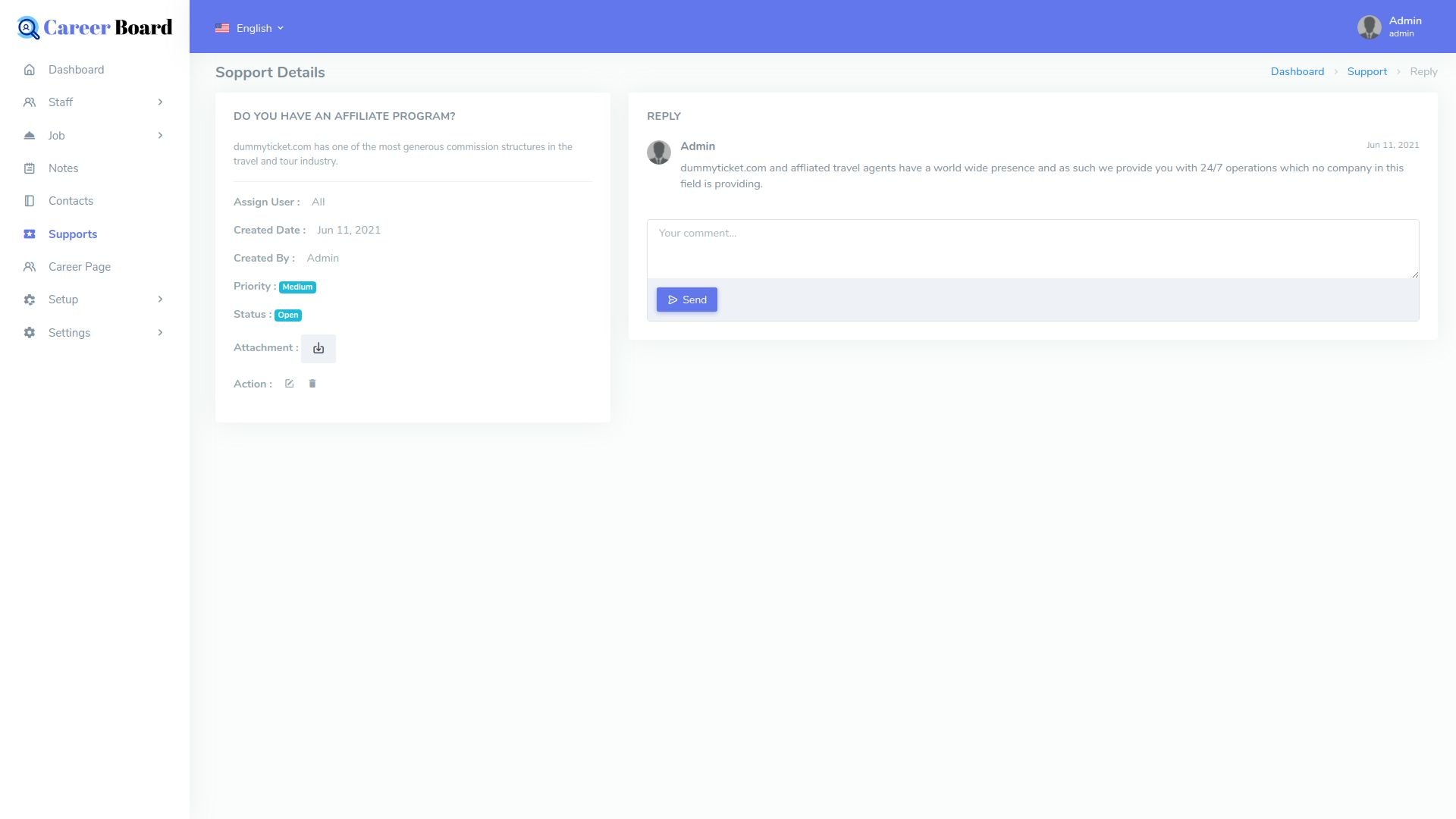The image is a screenshot of a professional webpage titled "Career Board," prominently displayed in purple and black text at the top alongside a blue magnifying glass icon. The navigation menu beneath the header includes various options: Dashboard, Staff, Job, Notes, Contacts, Supports (highlighted in purple indicating the active page), Career Page, Setup, and Settings.

In the main content area, the "Support Details" section is visible, featuring a query about an affiliate program. The displayed information includes:
- Question: "Do you have an affiliate program?"
- Response: "DummyTicket.com has one of the most generous commission structures in the travel and tour industry."
- Assigned User: "All"
- Created Date: "June 11th, 2021"
- Created by: "Admin"
- Priority: "Medium"
- Status: "Open"

Below this, functionality for adding attachments is provided, along with action buttons featuring a pencil (edit) and a garbage bin (delete) icon.

Further down, in the "Reply" section, the admin replies: "DummyTicket.com and affiliated travel agents have a worldwide presence, and as such, we provide you with 24-7 operations, which no company in this field is providing." This reply is dated June 11th, 2021.

At the bottom, there is an interface that allows users to respond with comments. This includes a "Reply" text entry field and a prominent purple "Send" button. The overall page design features a combination of a purple header, white content areas, and gray background elements, providing a clean and organized user interface.